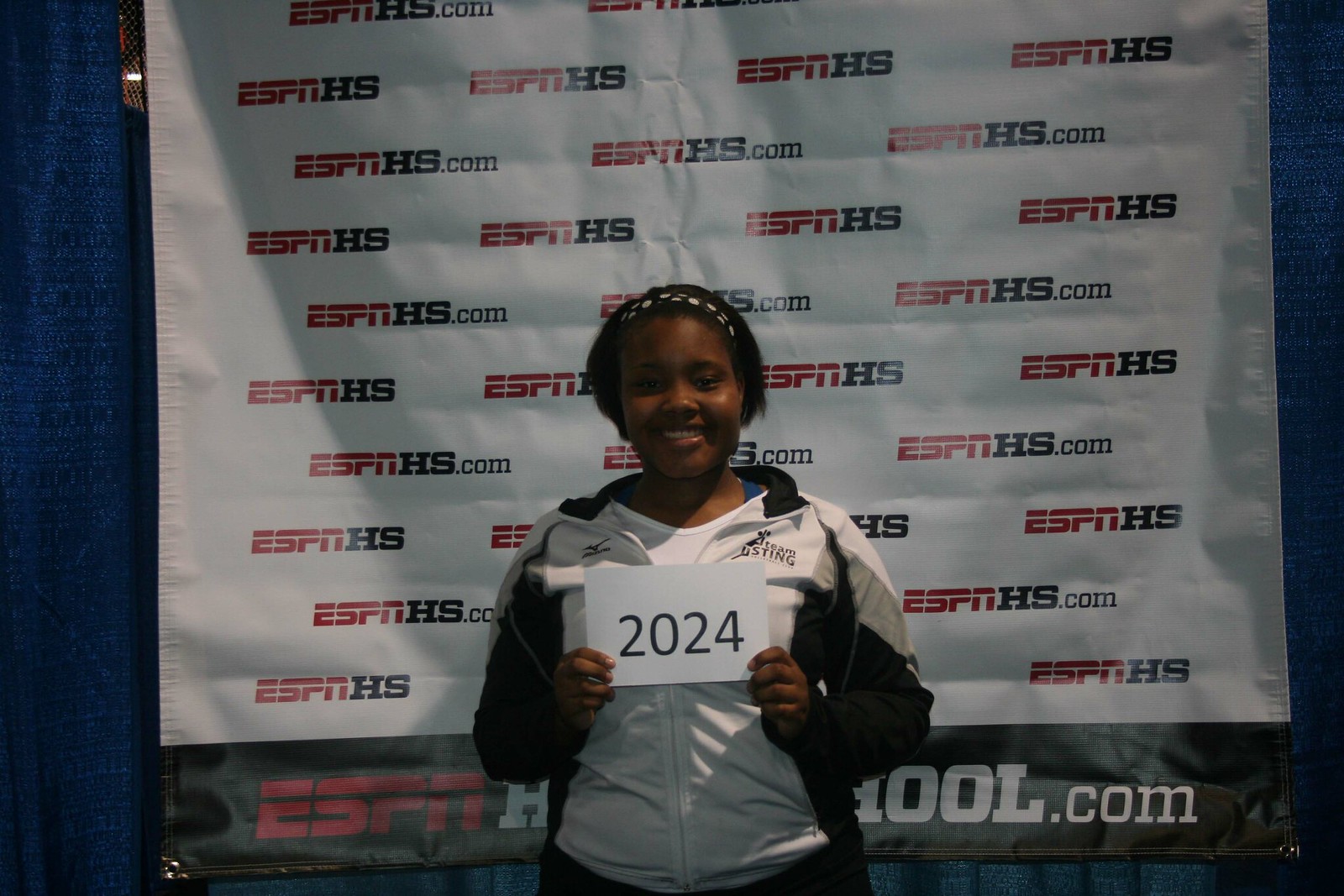This photograph captures a young girl of African descent standing proudly in front of a white banner with alternating horizontal and vertical text reading "ESPNHS.com" in red and black. The banner, nailed or stapled to a wall adorned with blue curtains on either side, features a black stripe running along the bottom. The girl is seen from the waist up, facing the camera, and smiling with her mouth open, revealing the top row of her teeth. She has short black hair pulled back with a white headband. She wears a white T-shirt underneath a black, white, and gray zip-up jacket. In both hands, she holds up a white, horizontal, rectangular sign in front of her chest, which has "2024" typed in black letters. The overall atmosphere suggests a sense of pride and achievement, possibly related to a sporting event or a school activity.